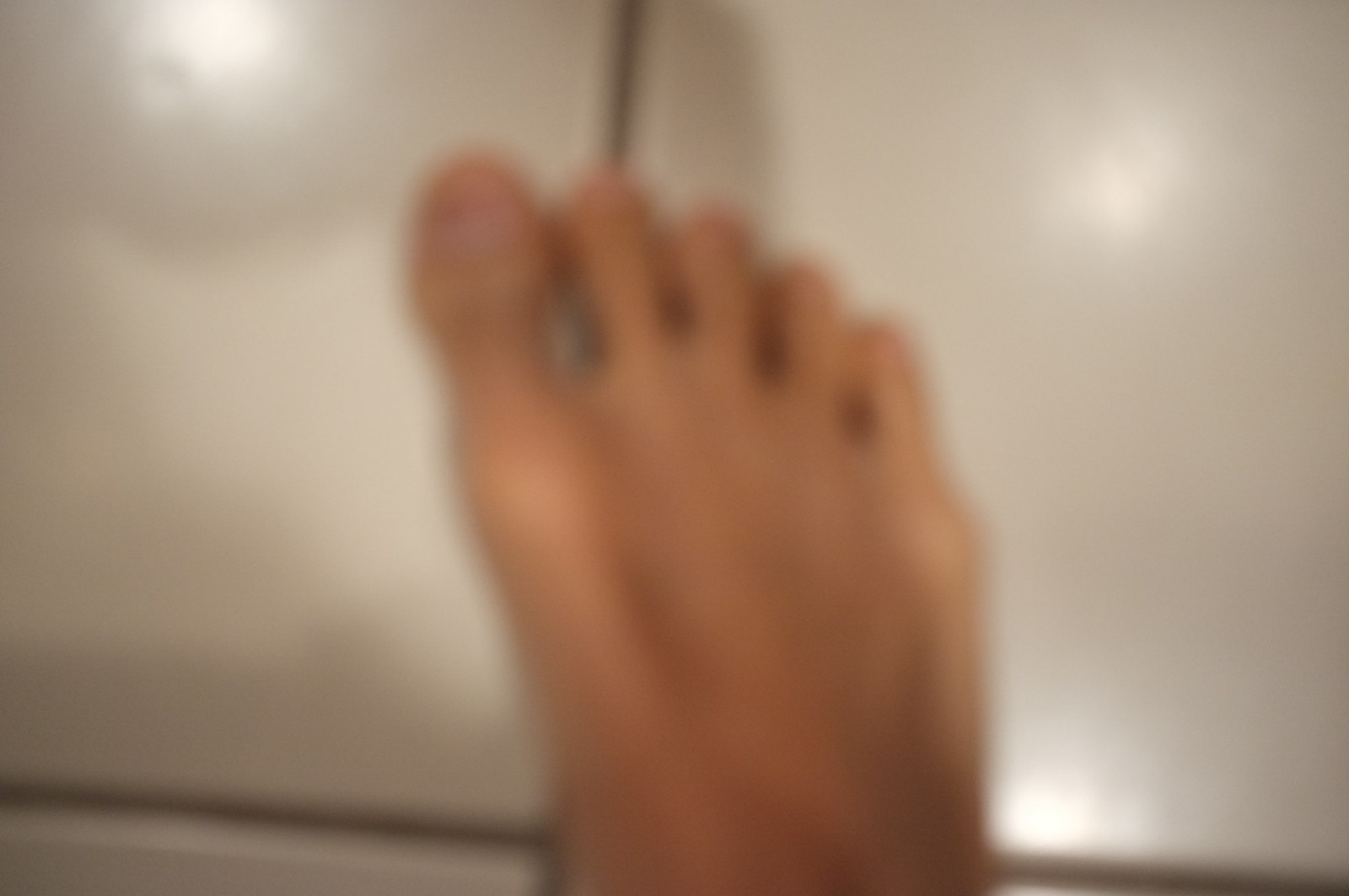In this blurry image, a human foot with a fair complexion rests on a white tile floor intersected by darker grout lines. The foot, positioned centrally, obscures the perpendicular junction of the tile lines near the bottom center of the photograph. Only the tops of the toes are visible, while the ankle and heel extend out of frame, out of sight. Though the toenails seem unpainted, the image's blurriness prevents clear discernment of finer details. Prominent bones suggest that the person may be quite thin.